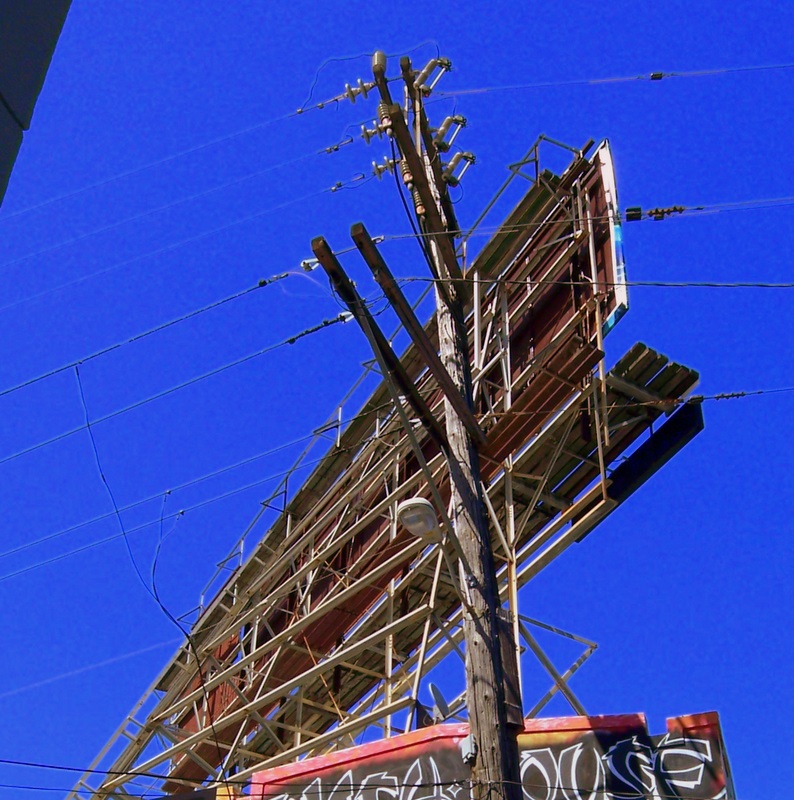This is a close-up, color photograph capturing the intricate details of urban infrastructure. Dominating the foreground is a very large wooden utility pole, bristling with multiple power lines extending in various directions. The background is strikingly vivid, featuring an almost surreal cyan-blue sky that contrasts sharply with the earthy texture of the wooden pole and the metallic gleams of the wires.

In the middle ground, there's a partial view of the backside of a billboard, revealing its steel framing and a wooden platform, likely used by workers for installing or changing advertisements. Adjacent to this, a streetlight juts into the frame, adding another layer of urban visual complexity.

Additionally, a sign is visible that reads "House" in a stylized, Asian-inspired font. The text is black, boldly outlined in white, and further accented with a red border, making it stand out prominently against the electric blue sky. The combination of these elements paints a detailed, lively portrait of a typical cityscape, rich with utility and character.